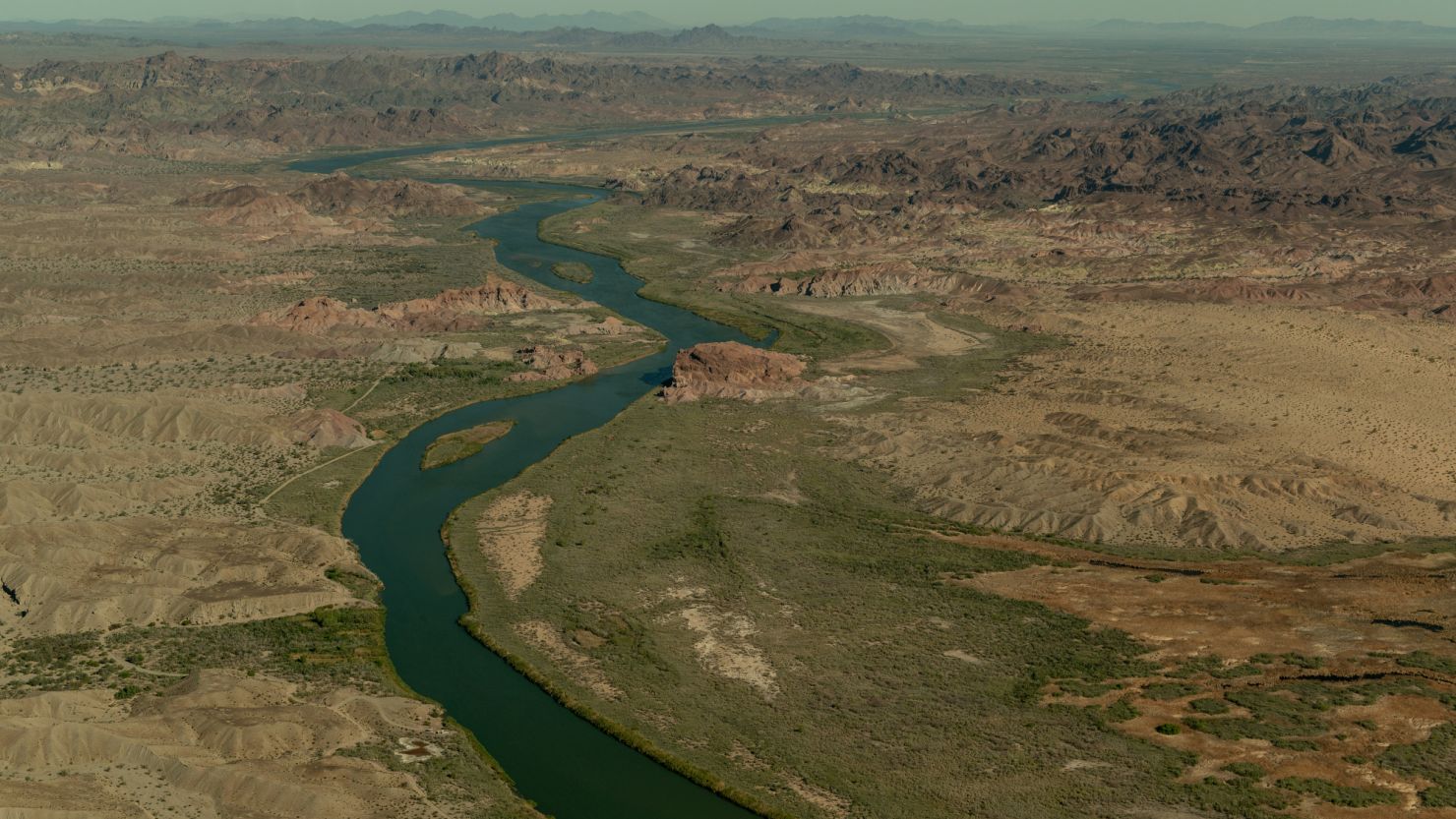The aerial shot captures a diverse landscape transitioning from desert to plains with varying hues of green and brown. Dominating the center of the image is a twisting river that starts at the bottom center, meanders slightly right, traverses through small islands, and then zigzags diagonally upward before veering left and concluding its visible path far to the right. The river itself is a thin blue line, contrasting sharply against the surrounding terrain. On the right side, a stretch of desert gradually becomes greener as it approaches the left. The left side of the image features plains, with patches of grass and bushes scattered throughout. In the distance, the landscape appears dotted with sparse trees and mountains, adding depth to the scene. The entire view, likely captured by a drone, showcases a harmonious blend of natural elements under a clear blue sky.